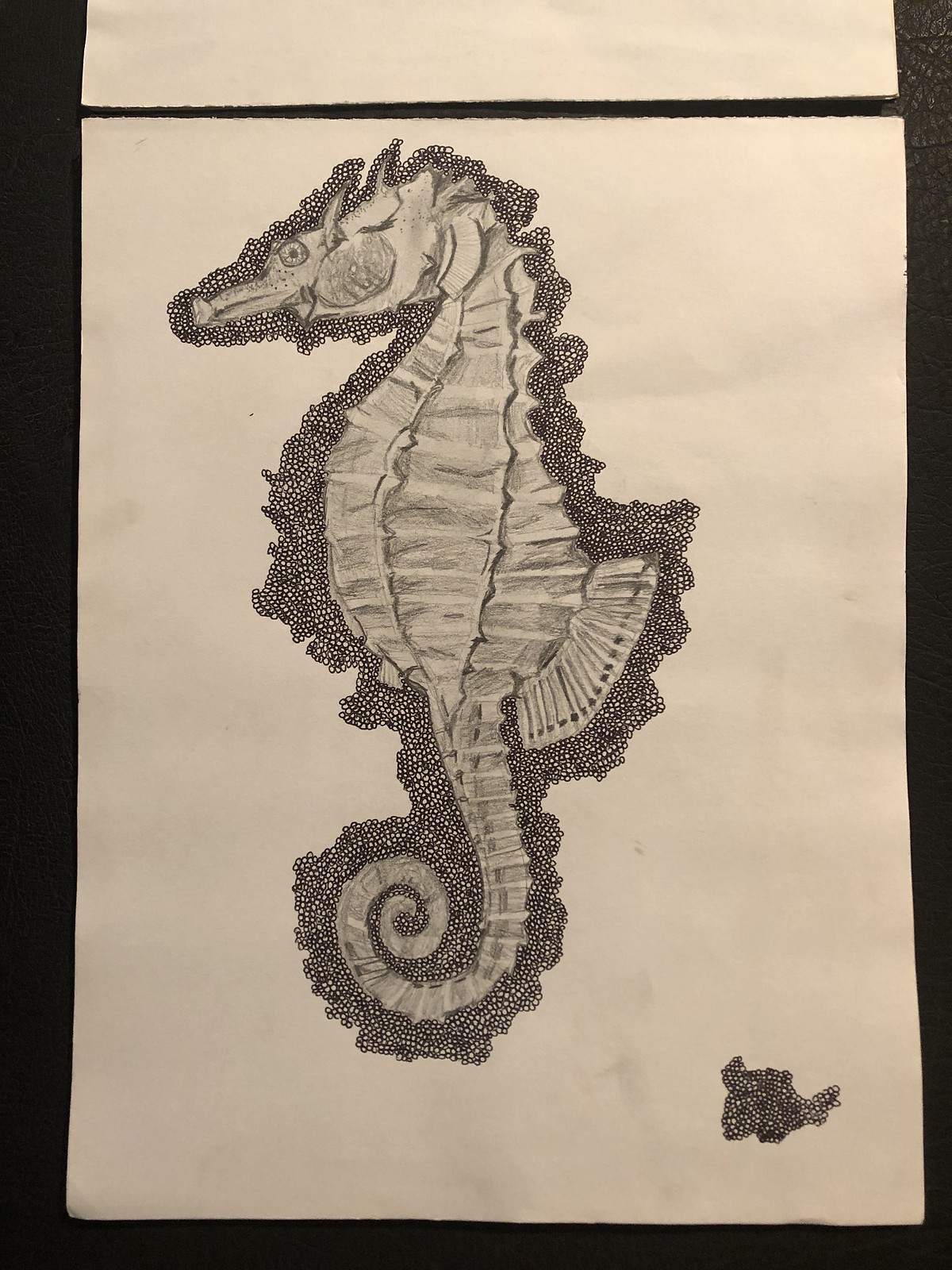This is a detailed photograph of a drawing that features an imaginative creature resembling a giant seahorse. The creature is depicted in shades of gray, black, and white, and stands imposingly tall. Its face is a fascinating blend of dragon and seahorse characteristics, with one visible eye and a prominent snout. The body of the creature is adorned with intricate scales and various lines that add to its textured appearance. It is outlined in a combination of black and white dots, adding a striking contrast to its form. Notably, the tail of the creature is elegantly curled at the end. The drawing is rendered on a pristine white sheet of paper, with a blank sheet positioned above its head, possibly indicating additional space for artistic expansion. At the bottom of the image, towards one side, a distinct black blob adds an element of mystery to the overall composition. The quality of the photograph is crystal clear, capturing every fine detail of the intricate drawing.